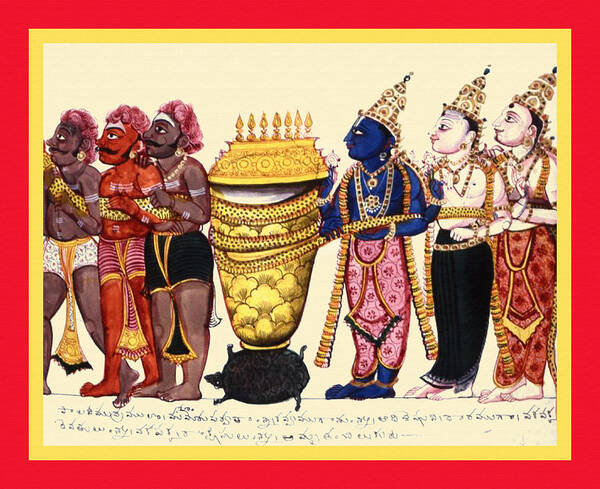The image depicts a vibrant, detailed poster featuring six Indian characters arranged in a traditional Indian style, all facing left. Each character, turned slightly with their left sides toward the viewer, is adorned in traditional Indian garb, with three men positioned on each side of a central golden urn. The three on the left display varied skin tones, including brown, red, and dark blue, the latter who notably wears pink pants. The other two characters flanking the central figure are paler in complexion. The urn, highlighted by lit candles adorning its top, rests on a base supported by what appears to be a black turtle. This turtle lies on its side, adding a unique element to the composition. Beneath the characters' feet and the urn, handwritten text in Hindi is visible, contributing to the traditional and cultural aesthetic of the poster. The scene is rich with colors and portrays a blend of human and seemingly supernatural elements, showcasing a dynamic interplay of vibrant and diverse artistic expressions.